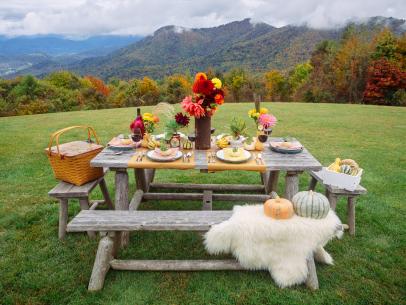This photograph captures an idyllic outdoor setting featuring a gray wooden picnic table on a lush, green grassy field. At the center of the picnic table is a vibrant bouquet of brightly colored flowers, including shades of pink, red, and yellow. There are six place settings evenly distributed around the table, each adorned with floral decorations and bright yellow placemats. To the left, a golden wicker picnic basket rests on one of the benches, while in front, the closest bench hosts a piece of white fur topped with two pumpkins—one traditional orange and the other a light green—adding a touch of fall's charm.

The background reveals a stunning autumn landscape with a line of colorful trees, displaying a spectrum of green, red, and brown leaves signaling the change of season. Beyond the tree line, green and brown mountains rise, their peaks softly obscured by a layer of fluffy white and gray-tinged clouds or possibly mist. Further accentuating the cozy outdoor scene is a smaller, children's chair positioned to the right of the bench, adding a feeling that this setting is ready to welcome guests of all ages.